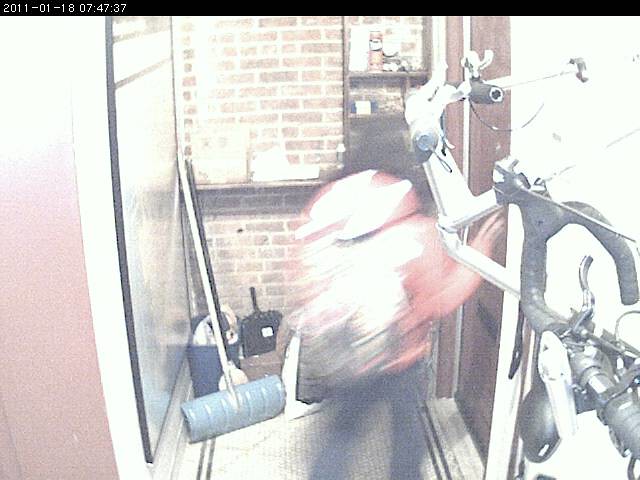A blurry photograph captures the entryway of a building. At the center of the image, a person with long dark hair is seen wearing a red puffy coat, jeans, and a tan backpack, as they extend their hand towards a door on the right. To their left, a shovel is propped against the wall, revealing its back. A brick wall stands in the background, adorned with brown shelving and various items. The left side of the photo shows a large poster on a coral-painted wall. A woven rug with long black vertical lines lies on the floor. To the right, part of an exercise machine is visible. The upper left corner of the photograph displays a timestamp: "2011-01-18 07:47:37."